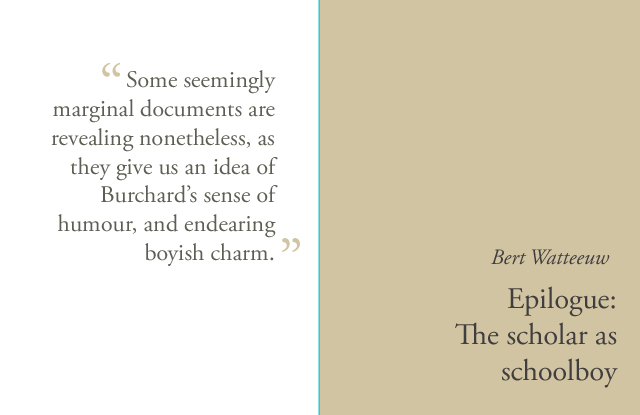The image is designed as a minimalist book cover divided into two halves. The left half features a white background with a quote in dark brown text, encased in light brown quotation marks. The quote reads, "Some seemingly marginal documents are revealing nonetheless, as they give us an idea of Bertrard's sense of humor and endearing boyish charm." A thin blue line vertically divides the image. The right half has a light brown background. In the lower right corner, in black text, is the author's name "Bert Latou," and below it, the book's title, "Epilogue: The Scholar as Schoolboy," presented in a stylish, minimalistic manner.